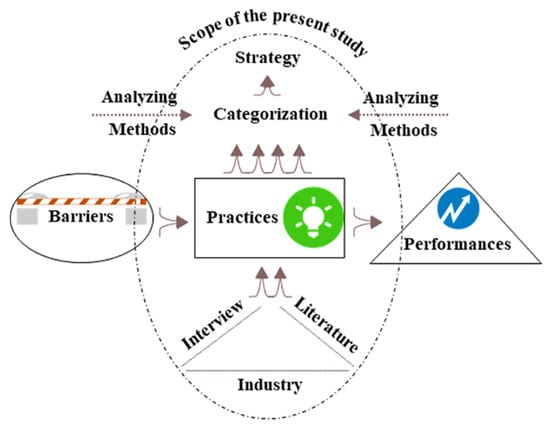The image is a detailed black-and-white diagram labeled "Scope of the Present Study" at the top in an arch. It features a broken oval shape that outlines the primary elements of the study. At the top of the oval is the word "Strategy," followed by "Categorization" beneath it. From the left and the right, "Analyzing Methods" point inward towards "Categorization." At the center of the diagram, a box labeled "Practices" contains a green circle with a white light bulb icon. Arrows point from "Practices" to various sections: leftward to "Barriers," rightward to "Performances," which is symbolized by a blue circle with a zigzag line, and downward to "Interview" and "Literature." At the very bottom, "Industry" is placed, connected via two upward-pointing arrows. The diagram visually connects these concepts with directional arrows, illustrating their interrelationships within the study's scope.